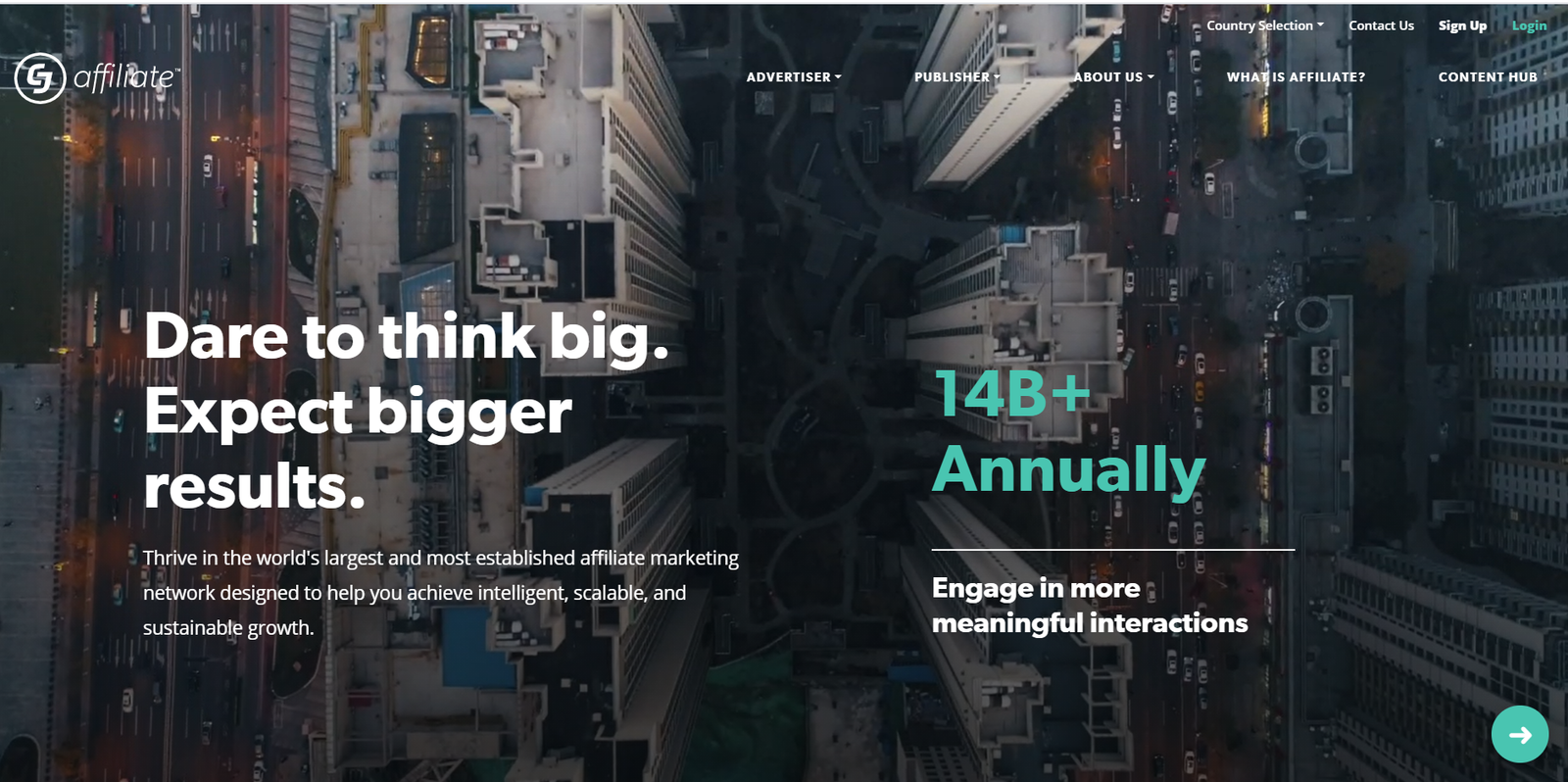The image depicts the landing page of the CJ Affiliate website. Prominently positioned in the upper left-hand corner is the CJ Affiliate logo. The central navigation bar includes links to key sections: Advertiser, Publisher, About Us, What is Affiliate, Content Hub, Login, Sign Up, Contact Us, as well as an option for Country Selection.

Dominating the visual backdrop is a sprawling, high-density urban landscape with numerous high-rise apartment buildings and a network of highways, evoking a "concrete jungle." The bustling cityscape suggests a thriving hub of activity and connectivity.

Overlaying this urban scene, the text—rendered in white and light sea green—emphasizes the platform's promise and capabilities. It highlights CJ Affiliate's achievements of over $14 billion in annual transactions, encouraging users to "Engage in more meaningful interactions," "Dare to think big," and "Expect bigger results." The text ultimately underscores the platform's commitment to enabling users to thrive within the world's largest and most established affiliate marketing network, designed to facilitate intelligent, scalable, and sustainable growth.